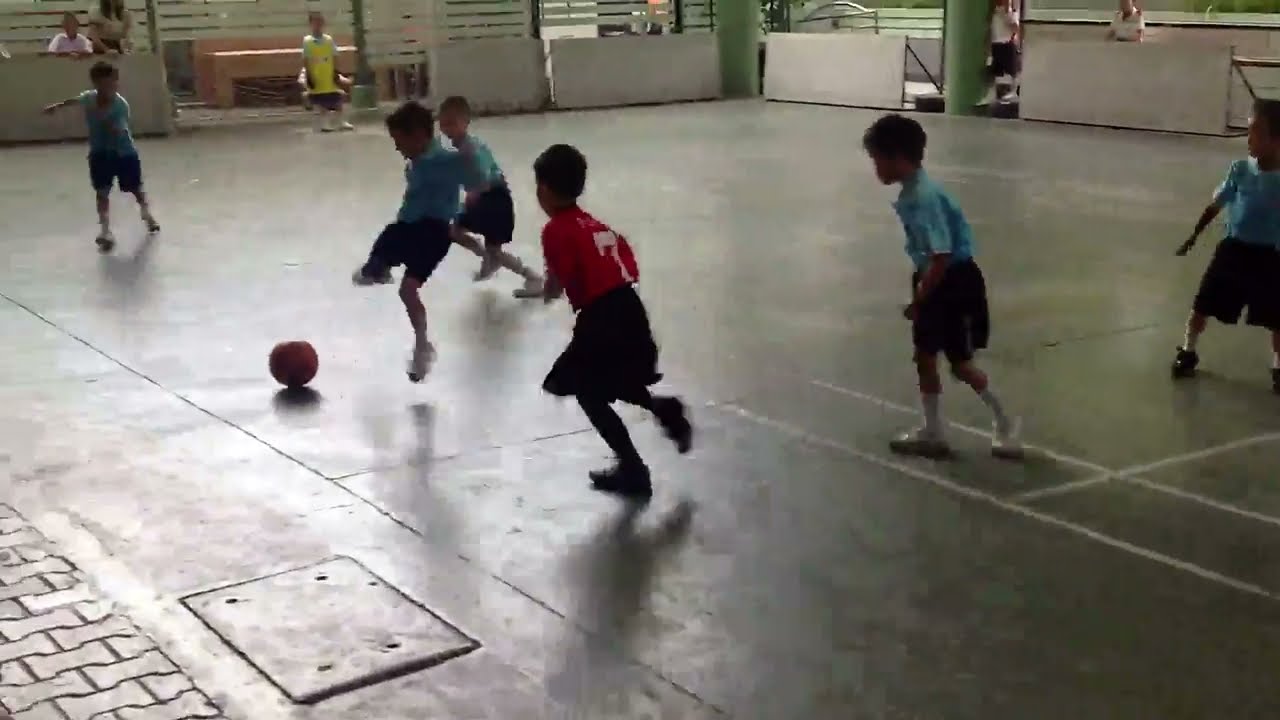In this lively image taken inside a gymnasium, six or seven children are energetically playing soccer on a hard surface, presumably concrete. The scene unfolds with vivid action as one boy, clad in a red jersey and black shorts, is captured mid-air, poised to kick the ball. Surrounding him are other children, some in light blue jerseys and navy blue shorts, attentively watching the dynamic moment. On the sidelines, a boy in a yellow jersey sits on a bench, while a few spectators sit on bleachers in the background, observing the game intently. The gymnasium features white panels acting as barriers to keep the ball within bounds, and through some partitions, a glimpse of an outdoor grass field is visible. The children, approximately seven or eight years old, exhibit the vibrant spirit of youth learning the cherished sport of soccer.